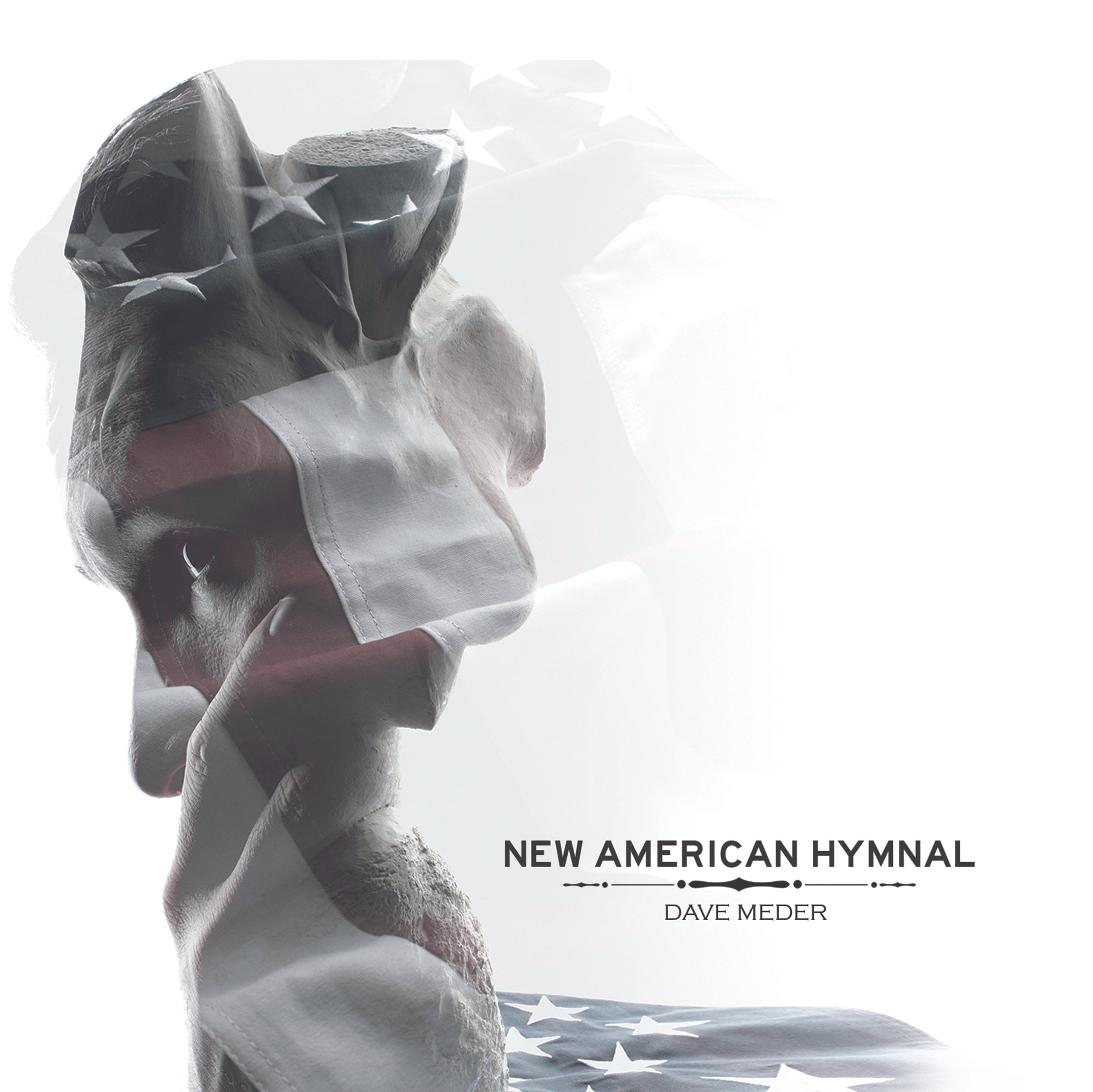The image is a manipulated photograph featuring a silhouette of a man's face, seen in profile, with his hand over his chin in a contemplative pose. His face is partially wrapped in the American flag, with blue and white stars overlaying his forehead and red and white stripes crossing his profile. There's a subtle hint of a rock or cliff structure beneath the flag and face overlay. To the right of this composition, the words "New American Hymnal" are prominently displayed, followed by a thin divider and the name "Dave Meador," indicating the likely creator. The overall aesthetic of the image combines a grayscale palette with selective coloration of the flag, and the top portion appears intentionally broken or distressed.